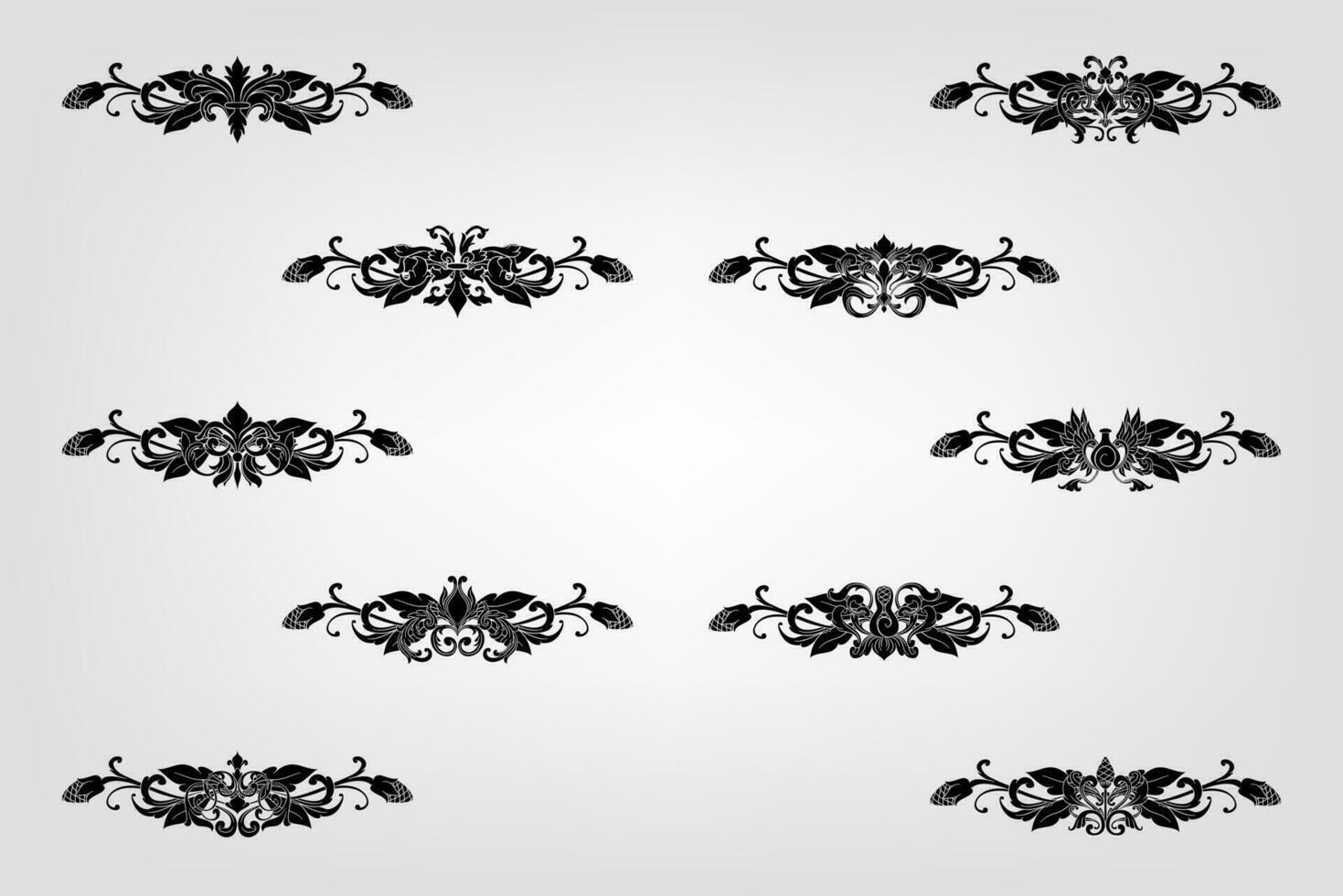The image displays a detailed black and white artwork set against a light gray background, arranged in a horizontal rectangular layout. Twelve intricate designs, each slightly varied but fundamentally similar, form an oval in the center. These designs feature a central rosebud encircled by four leaves, two on either side, entwined with vine-like stems. Some designs show additional elements like vases and diamond-shaped leaves. The patterns are symmetrically positioned with one in each corner and six in the middle, contributing to the overall sense of balance and artistry. The grayscale contrast highlights the delicate interplay between the floral and leafy components.